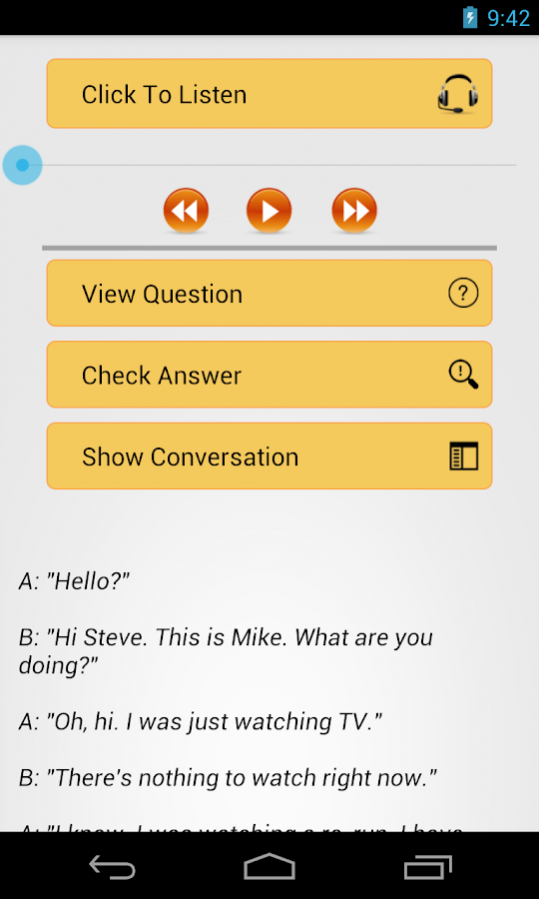This is a detailed screenshot of a mobile device interface. The layout includes a black header and footer, with a light gray background filling the rest of the screen. In the top right corner of the black header, there are blue icons and text. 

Centered in the body of the page is an orange rectangular object with a darker orange thin outline. On the left side of this rectangle, black text reads "Click to listen," accompanied by a headset icon on the right side, casting a small gray shadow underneath it.

Below this orange element runs a thin medium gray line extending almost entirely across the page. Positioned on the left side of this line is a small blue dot, surrounded by a light blue translucent circle.

Underneath this line and centered on the page are three orangish-yellow orbs. Each orb contains a white icon: the left orb features two left-pointing arrows one after the other, the right orb mirrors this with two right-pointing arrows, and the center orb displays a slightly larger single right-pointing triangle.

Below the orbs lies another medium-width medium gray separator line running nearly the width of the page. Following this line are three similarly styled orange rectangles stacked vertically. Each rectangle includes black text on the left and corresponding black icons on the right. From top to bottom, the labels read "View Question," paired with a question mark icon encircled; "Check Answer," paired with a magnifying glass containing an exclamation point inside it; and "Show Conversation," paired with relevant iconography.